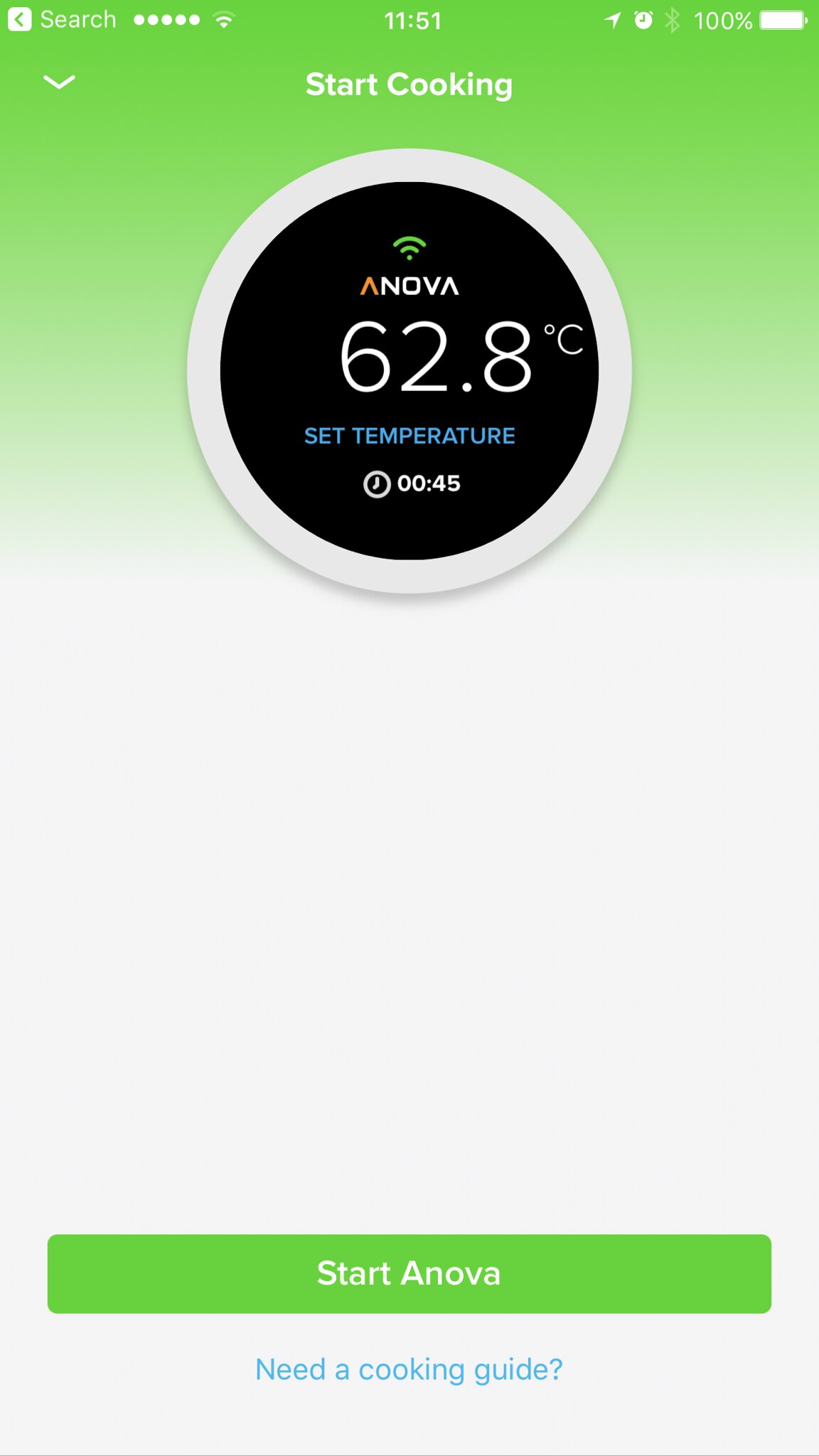The image is a screenshot taken from an iPhone, as indicated by the typical iPhone status bar at the top showing the time as 11:51, 100% battery life, Wi-Fi connectivity, and cellular signal strength. The screenshot captures an app interface, prominently featuring the text "Start Cooking" at the top.

The app appears to be related to cooking, likely by an advanced kitchen appliance brand, as inferred from the name “Anova” displayed at the top-center. The brand name features a stylized design, with "A" in orange and the rest of the letters in white. Above the brand name, there is a green Wi-Fi symbol indicating connectivity.

Beneath the "Start Cooking" text, the current temperature is displayed: 62.8 degrees Celsius, with the label "Set temperature" written in blue right below it. Directly underneath this, there is a timer showing "00:45" (45 seconds).

At the bottom of the screen, a long green button displays the text "Start Anova," suggesting that pressing it initiates the cooking process. Below this button, there's a blue text link that reads "Need a cooking guide," inviting users to access additional resources. 

The background of the app is visually divided: the top section is green, while the remainder of the background is white, ensuring a clean, visually organized interface.